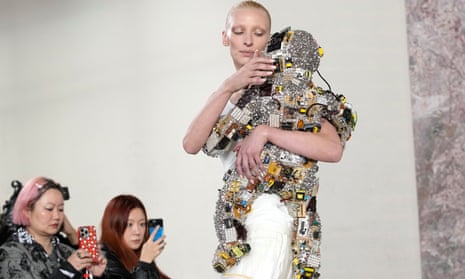In a stylish fashion setting, a European model with pale, peach-white skin, dressed in a pristine white outfit, is tenderly cradling a young child. The model's hair, possibly short or slicked back, is not visible. She gazes down at the child with a nurturing expression, holding the toddler securely in her arms. The child is adorned in a striking and elaborate metallic outfit, primarily silver and yellow, resembling a futuristic cyborg or cosmonaut. The suit includes intricate wiring from the headgear to the shoulder, enhancing the high-tech appearance. The baby's face is not visible, adding to the mystique. In the background, two women, one with dark brown hair and the other with pink hair, are seated and taking pictures with their blue and red cell phones, respectively. Their presence underscores the attention and interest in the scene, capturing the blend of humanity and robotic aesthetics.